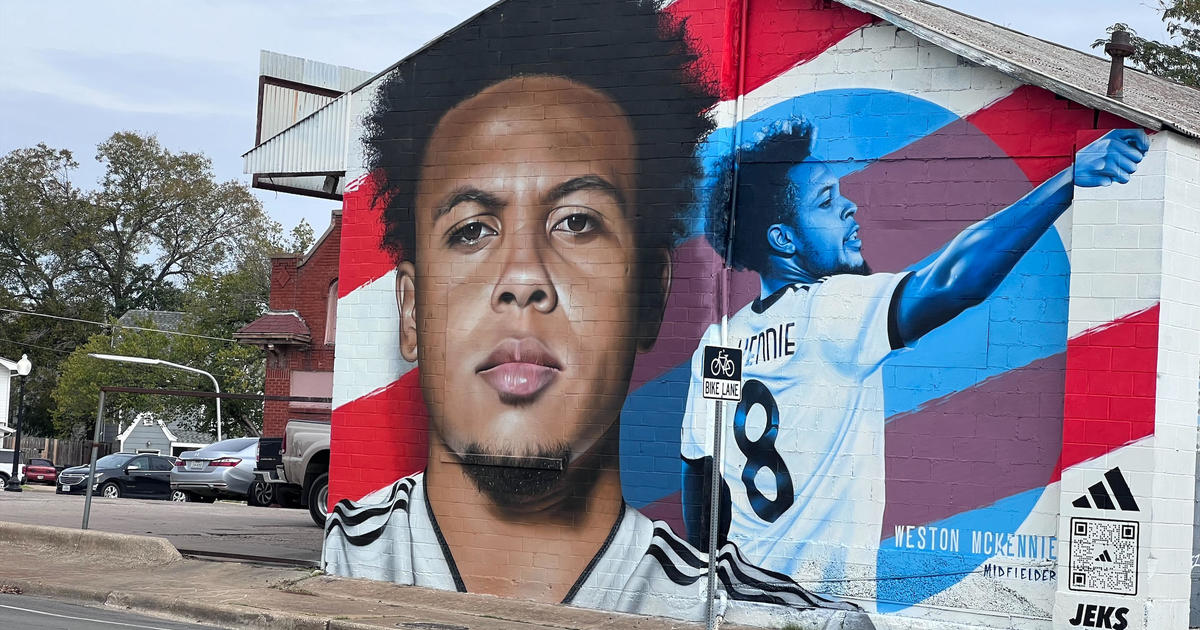The image showcases a vibrant mural on the side of a building, prominently featuring African-American soccer player Weston McKennie. The athlete's portrait occupies a large portion of the mural, displaying a serious expression as he looks forward, juxtaposed with another image of him, seen from behind, smiling and raising his hand. His jersey, marked with the number 8, is rendered in a blue tint with a circular blue background. Behind him, the American flag adds a patriotic touch. An Adidas logo and a QR code are also incorporated into the mural, indicating it might be a sponsored piece. The mural is in a setting that includes a glimpse of a sidewalk, a bicycle lane sign, and a parking lot with a few cars. In the background, some trees and parts of other buildings can be seen, suggesting an urban environment.